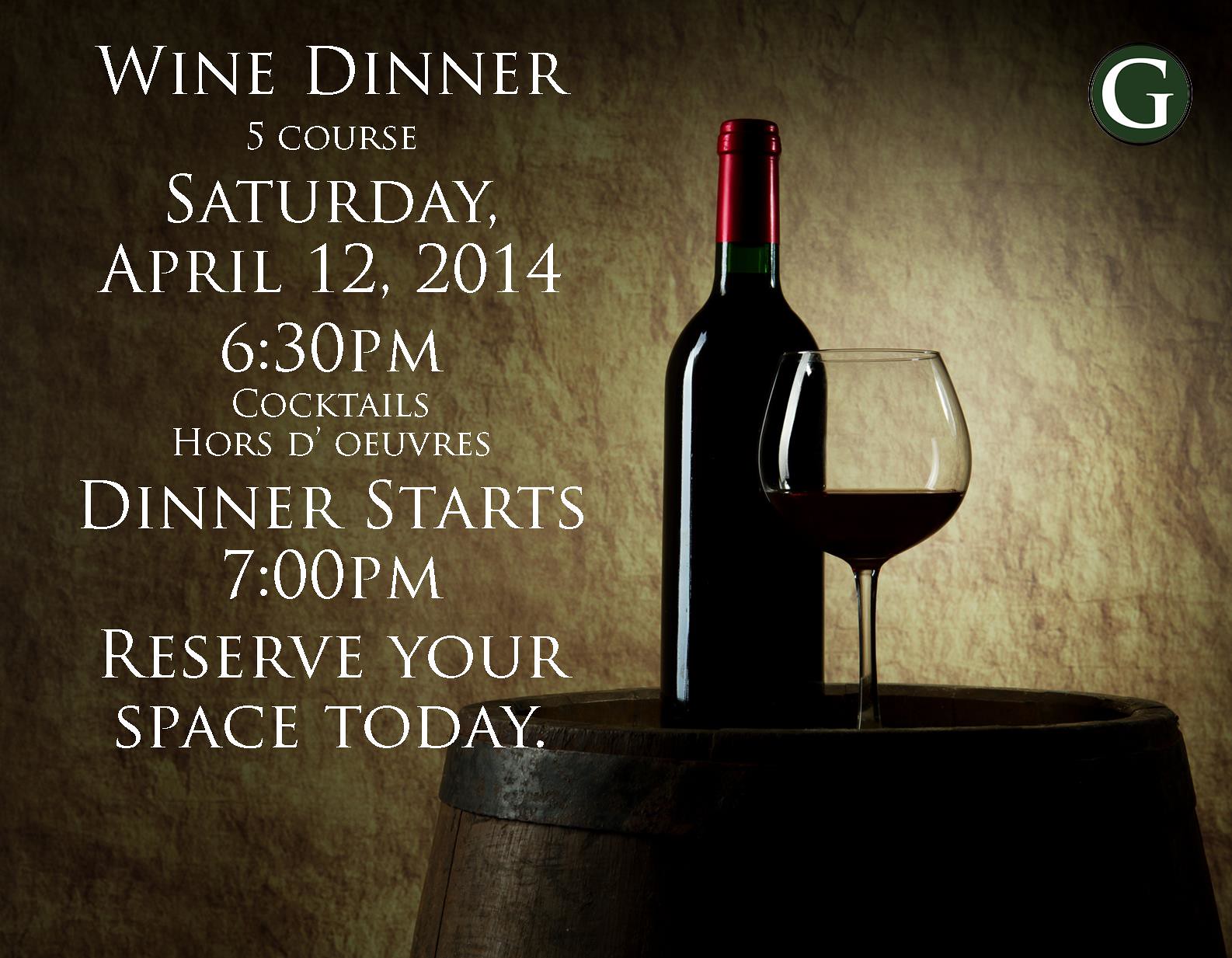The image is a dark-toned promotional poster with a brown or beige tint, advertising a wine dinner event. On the left side, white text in a column format reads: "Wine Dinner, 5 course, Saturday, April 12th, 2014, 6:30 p.m. Cocktails, hors d'oeuvres, dinner starts 7 p.m., reserve your space today." At the right center of the picture, a wooden whiskey barrel hosts a dark wine bottle with a red cap and neck. Alongside the bottle, a wine glass is partially filled with a dark fluid. The background features a brownish stone wall, with a green circle containing a white letter "G" in the upper right corner.